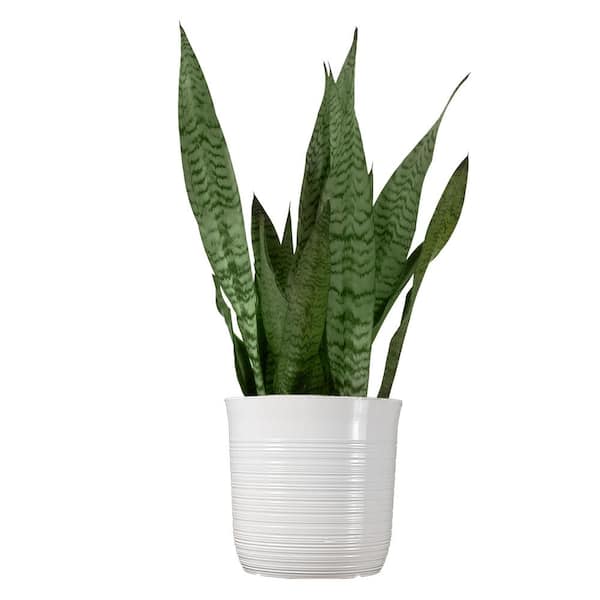This image features a healthy, vibrant plant set against a solid white, text-free background. The plant is housed in a white ceramic pot that has horizontal lines adding a touch of texture and design, though the rim at the top is smooth. The plant itself appears to be a snake plant, characterized by its tall, vertical leaves that range in length. Each leaf showcases a unique pattern of varying shades of green, with darker green forming an upside-down V pattern along the leaf surfaces. The leaves are primarily vertical, though some deviate slightly to the sides, and they taper to sharp points. In total, there are about 15 to 20 leaves, creating a dense and lush display. The overall appearance is one of a well-maintained and aesthetically pleasing plant that could easily complement indoor decor, such as in a living room or backyard setting.